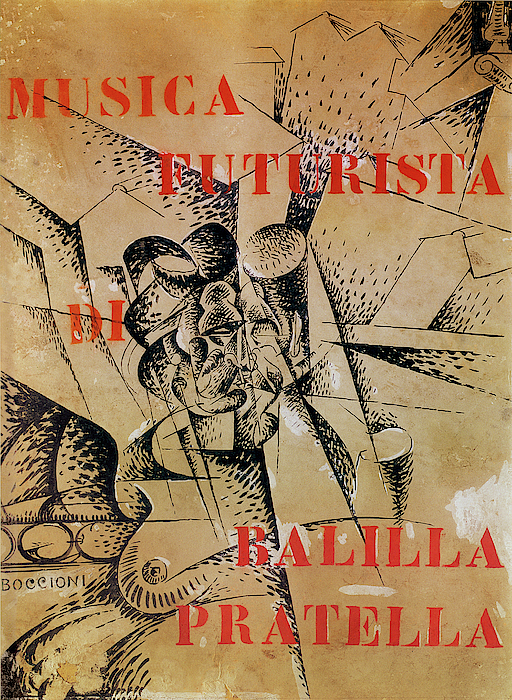The image features a piece of artwork, potentially a book cover, showcasing an abstract and geometric composition. The background is a dynamic blend of light brown and darker brown tones, intricately speckled with white. The central focus reveals an abstract, almost shattered-looking head outlined in black ink, resembling shattered glass in its composition. This head outline is very geometric and rough, showing discernible features like eyes and a nose despite its abstract nature. Scattered across the image are black dots and lines, which are complemented by striking red stenciled text. This text prominently displays the title "Musica Futurista," followed by the letters "D-I" and the name "Balilla Fratella" near the bottom right corner. Overall, the piece combines elements of futurist design and abstract expressionism, possibly promoting a music-related theme.